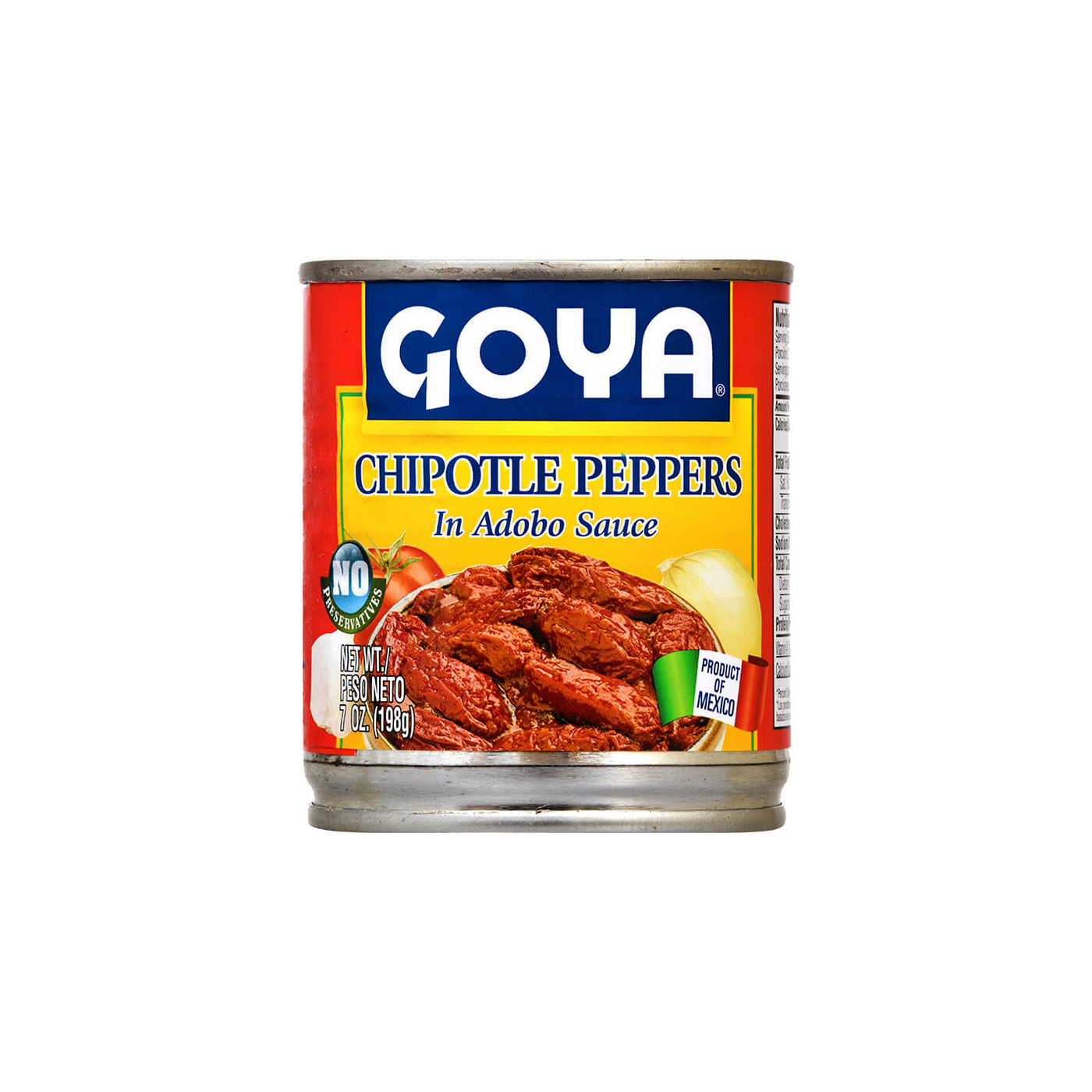This is a vertically rectangular, full-color photograph of a silver aluminum can of Goya Chipotle Peppers in Adobo Sauce, staged for promotional purposes. The can's label prominently features a blue rectangle at the top with "Goya" written in bold, white uppercase letters. Below it is a yellow box with "Chipotle Peppers" in large blue letters and "in Adobo Sauce" in smaller, italicized blue letters. The background of the label is red. An appetizing image of the red, wrinkly peppers in a white bowl is central on the label, flanked by a tomato on the left and an onion on the right. At the bottom of the label, a banner with the Mexican flag reads "Product of Mexico." To the left, it states "No Preservatives," and at the bottom left, it notes the net weight: "7 ounces (198 grams)." The right side of the can contains nutritional information, although it is not visible from this angle.